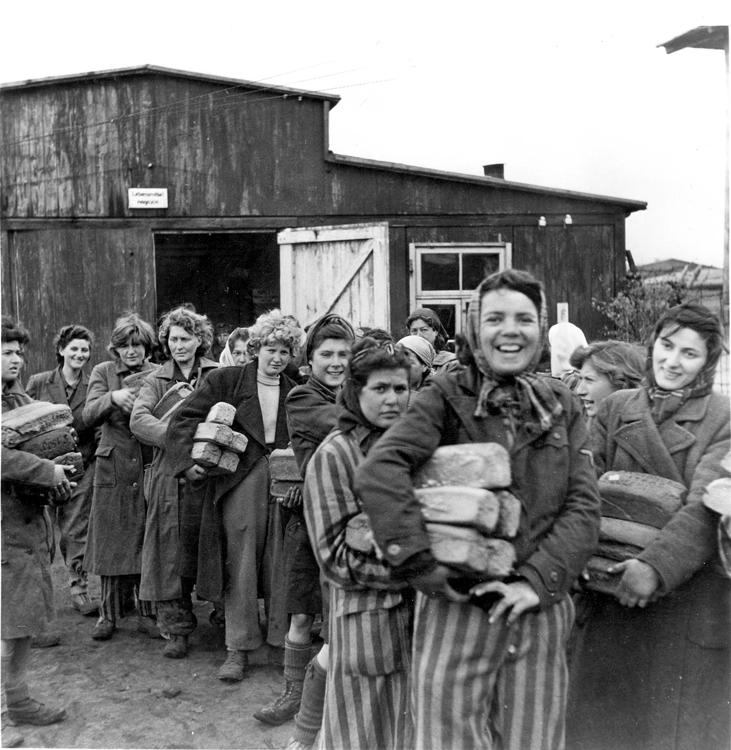In this black-and-white photograph, a line of women is standing in front of a large barn-like structure with an open door and a nearby window. The women are dressed in striped pants and dark coats, with many of them wearing fabric bonnets on their heads. They are carrying what appear to be large, square packages or possibly bread loaves in their arms. The women's expressions vary, with some smiling while others look serious. The attire and overall scene suggest an older time period, possibly the 1920s or during a wartime era, as they seem layered up as if it's cold outside. Despite the somber backdrop, the mixture of smiles and serious faces gives an ambiguous yet poignant atmosphere to the image.